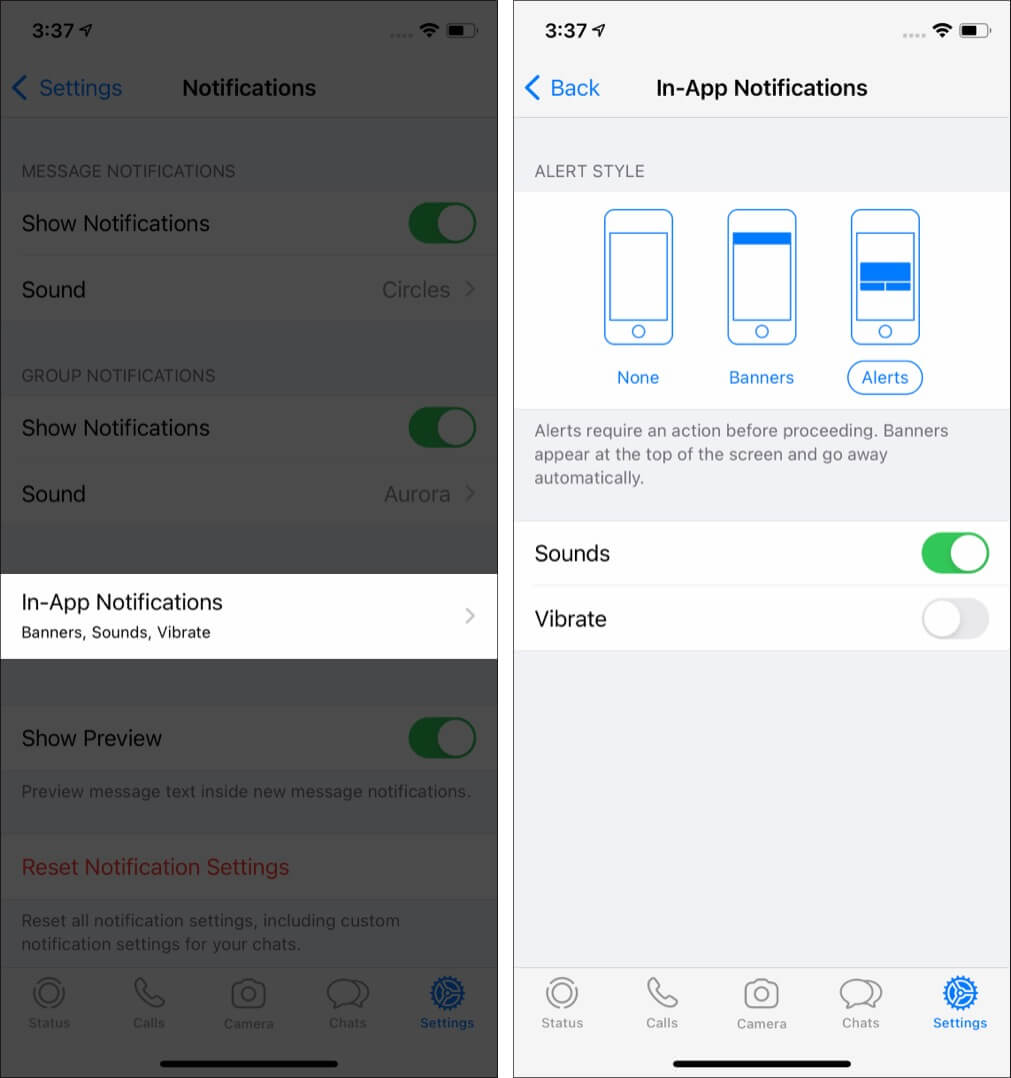The image features two split screenshots of mobile phone settings. On the left side, the screen displays general notification settings, while on the right, it showcases in-app notification settings.

**Left Screenshot - General Notifications:**
- The top bar features the title "Notifications" centered, accompanied by a settings button and a back arrow (<) pointing left.
- Below the title, the first category is "Message notifications":
  - It includes an option labeled "Show notifications" with a green toggle switch indicating it's enabled.
  - This is followed by a "Sound" setting, represented by the sound choice "Circles" and a forward arrow (>), suggesting more options are available upon tapping.
- The next category is "Group notifications":
  - It similarly has "Show notifications" with a green toggle switch turned on.
  - The "Sound" choice under this category is "Aura," also accompanied by a forward arrow (>).

**Right Screenshot - In-App Notifications:**
- The screen title "In-app notifications" is displayed within a white rectangular box, specifying that it includes banners, sounds, and vibrations.
- At the top left, a back button with a less-than sign (<) allows users to return to the previous screen.
- Below the title, there is a section for "Alert styles," illustrated with three icons representing different notification types:
  - "None" (depicted with a blank cell phone),
  - "Banners" (showing a mobile phone with a small overlay),
  - "Alerts" (represented by a phone with a full-screen notification).

This detailed setup helps users customize their notification preferences for both general messaging and in-app alerts, providing clear and accessible control options.